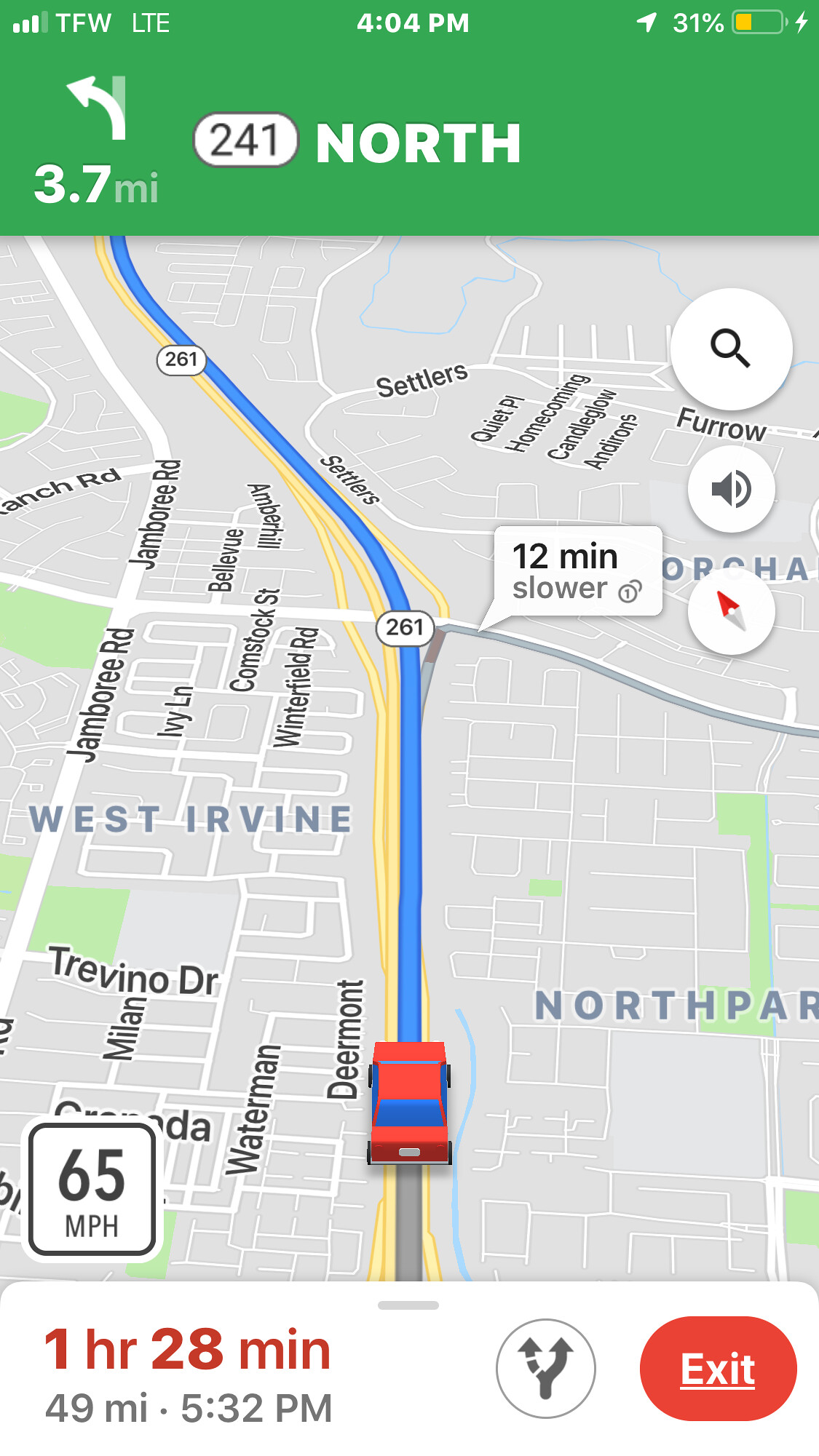A digital map display from a GPS navigation system shows the route for a car traveling on Highway 268, a 65 mph road. The screen reveals upcoming traffic congestion, which will delay the journey by approximately 12 minutes. Notable streets visible on the map include Trevino Drive, Jamboree Road, Settlers Furrow, and North Paw. The map indicates that the car is 3.7 miles away from the 241 North exit, which is the intended course. The final destination is 49 miles away, estimated to take 1 hour and 28 minutes to reach. The time displayed on the screen is currently 5:32 p.m. An alert indicates the device's battery is at 31% charge. The top of the screen shows the connection status as "TFW LTE."